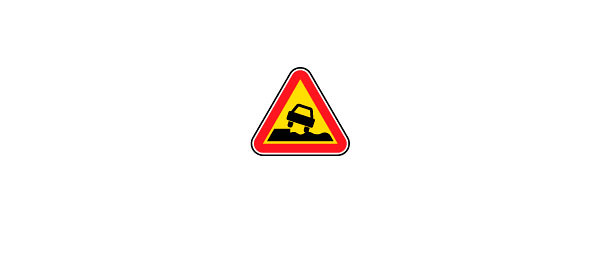The image depicts a triangular warning sign with a sleek black outline, enclosed by a wide red stripe. Inside the red triangle, a smaller, vibrant yellow triangle serves as the background for a silhouetted black car. The car, resembling a tilted sedan with two visible wheels and a rear window, is depicted climbing an uneven, rocky road. The entire scene is set against a stark white background, emphasizing the importance of the warning—drivers should proceed with caution due to the rough terrain ahead.